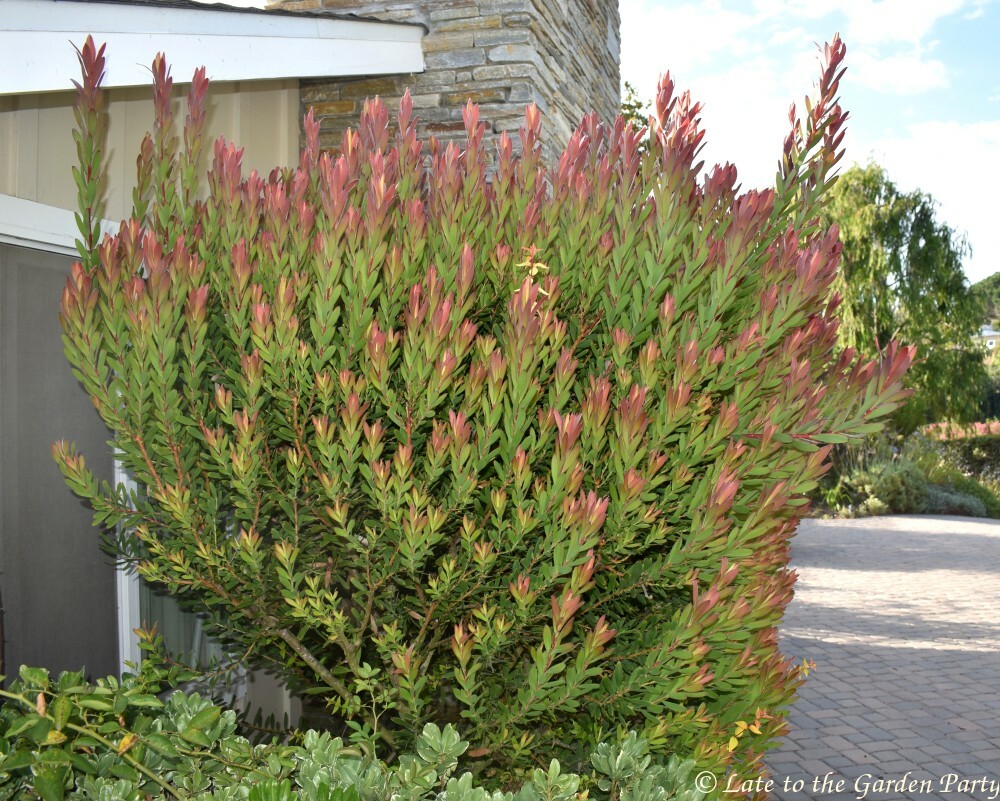This is a detailed photograph of a residential scene, prominently featuring a large, green and pink flowering bush. The bush is situated next to a gravel driveway and appears to be thriving with pink leaves clustering at the tips, giving an impression of flames or blossoms. To the left of the bush, the house's façade showcases screened-in windows with white paneling. Further in the background, additional trees provide a lush green backdrop. On the left side of the image, a brick building is partially visible, adding texture to the scene. Towards the bottom, another smaller plant with green and yellow tinges is visible. The image is copyrighted by "Late to the Garden Party", noted in the bottom right-hand corner.